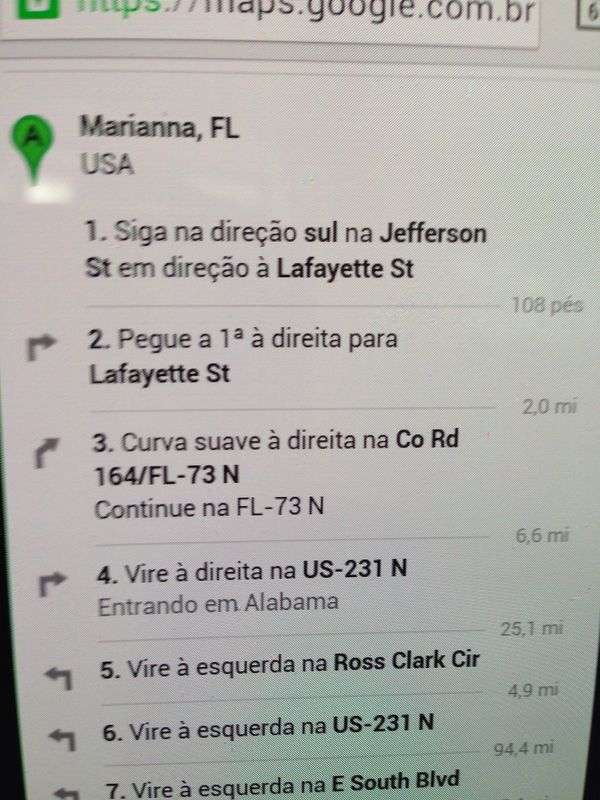Screenshot of navigation directions written in a foreign language, detailing a route that begins in Mariana, Florida, USA. At the top of the screenshot is a URL: "https://maps.google.com.vr," accompanied by a small green bubble with the letter "A" on a white background. 

The directions are as follows:
1. "Siga na dirasio suel na Jefferson Street" – Follow the straight path on Jefferson Street.
2. "Em dirasio a Lafayette Street, 108 Pes" – In the direction of Lafayette Street, for 108 feet, followed by a right turn.
3. "Two peg a one a dietre para Lafayette Street, two miles" – Continue to Lafayette Street for 2 miles, turning right again.
4. "Curva sabe e direte na County Road 164 FL 73 North" – Turn right onto County Road 164 (FL 73 North).
5. "Vera e direte en a US 231 North" – Turn right onto US 231 North.
6. "Vera a escuadrilla na Ross Clark CR" – Turn left onto Ross Clark Circle Road.
7. "Vera a escuadrilla na US 231 North" – Make another left onto US 231 North.
8. "Vera a escuadrilla na East South Boulevard" – Finally, turn left onto East South Boulevard. 

Each step is accompanied by respective directional arrows and distance indicators.